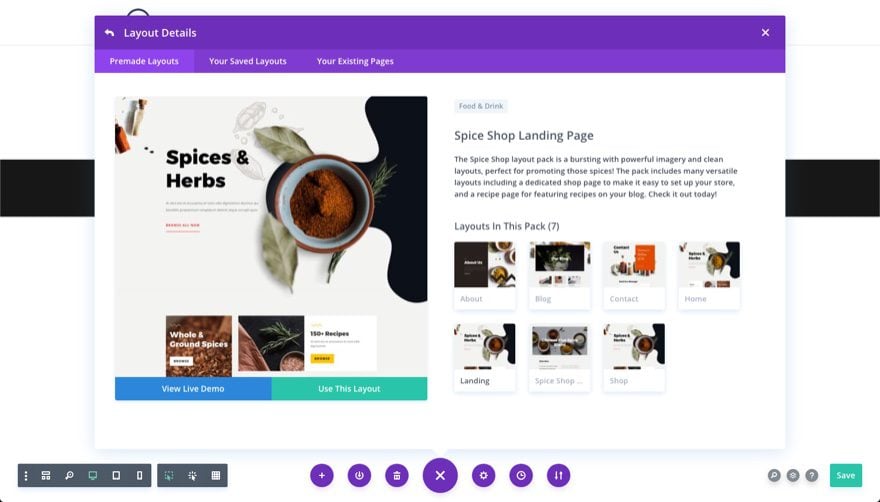This is a detailed screenshot of a webpage layout from a computer. The page features various elements that are cleanly organized for easy navigation. At the top, there is a prominent purple rectangular bar with white lettering that reads "Layout Details." Below this bar, there are three categorically structured sections: "Pre-Made Layouts," "Your Saved Layouts," and "Your Existing Pages."

Occupying the left half of the screen is an eye-catching image of a small jar filled with dark brown spices, accompanied by green leaves and a sprig of fresh herbs. Next to this image, the text "Spices and Herbs" is displayed, although the text directly beneath it is not clear in this screenshot. Below this, two distinct boxes are visible: one highlighting "Whole and Ground Spices" and the other emphasizing "150+ Recipes" alongside corresponding imagery of spices and greenery.

Towards the bottom part of this section, two vibrant buttons are presented: a blue button labeled "View Live Demo" and a green button labeled "Use This Layout."

On the right side of the image, the text "Food and Drinks, Spice Shop, Landing Page" is clearly visible, followed by a descriptive paragraph explaining the context or purpose of the layout. Just beneath this paragraph, there are two rows of navigation boxes. The first row includes "About," "Blog," "Contact," and "Home" buttons, while the second row consists of "Landing," "Spice Shop," and "Shop" buttons. Additionally, there are a set of icons located at the bottom, indicative of various computer functions.